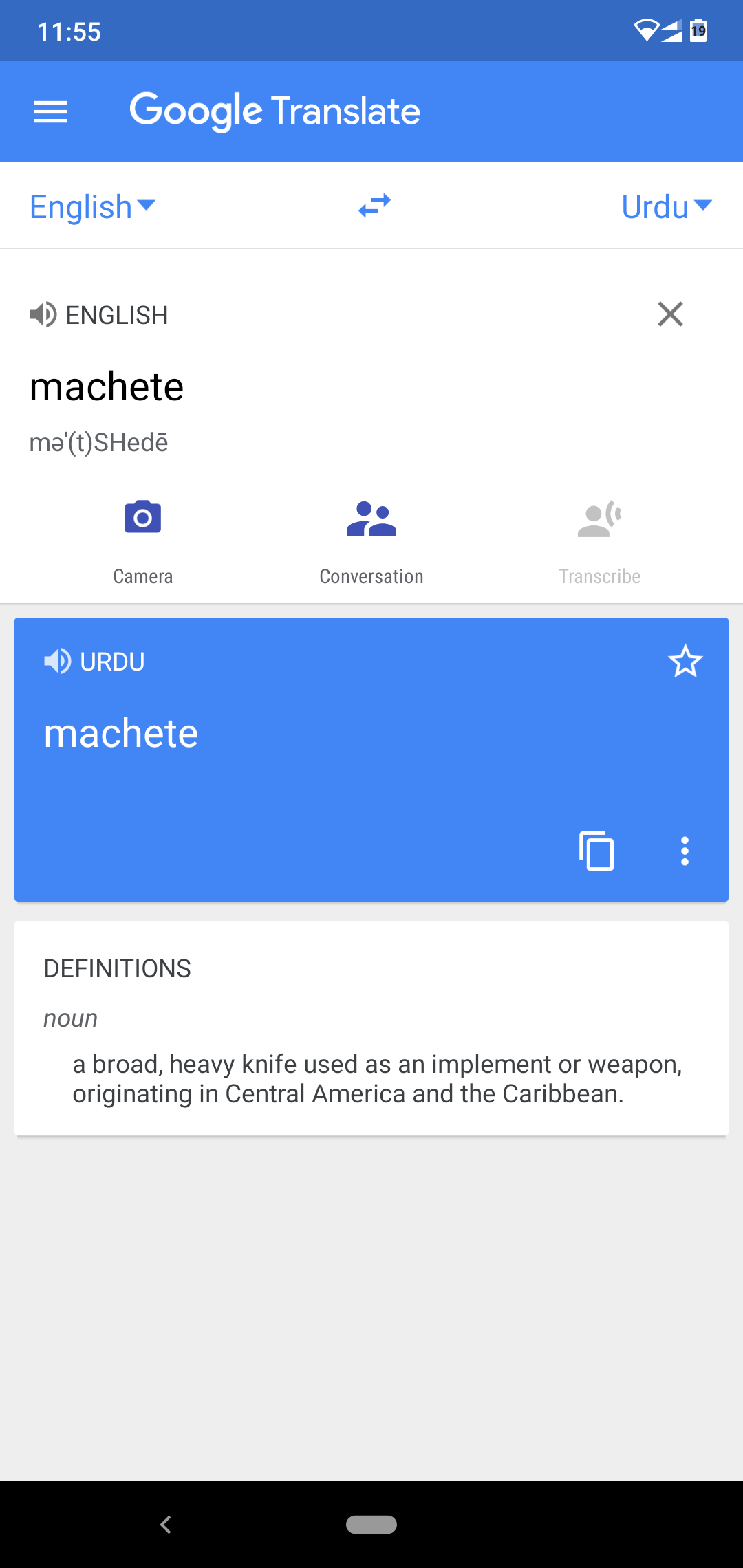A screenshot from an Android device displaying the Google Translate app is shown. The time at the top of the screen reads 11:55, alongside medium Wi-Fi signal strength, four bars of mobile data, and a battery indicator showing approximately 30% charge remaining. 

At the very top, a light blue header features a hamburger menu on the left and the title "Google Translate." Directly beneath, there's an input bar with drop-down menus for selecting the source and target languages, which are currently set to translate from English to Urdu. The input word is "machete."

Below the input bar, the translation section displays the word "machete" in both English and Urdu. A blue box labeled "Urdu" contains a speaker icon, suggesting that tapping it will play the word "machete" with an Urdu pronunciation. 

In the lower right corner of the translation section, there's a copy icon represented by two rectangles stacked on each other, a menu icon with three vertical dots, and a star symbol likely indicating a favorite option. Further down, the app provides the definition of "machete," labeled as a noun: "a broad, heavy knife used as an implement or weapon originating in Central America and the Caribbean."

The bottom of the screen features a black navigation bar with a return arrow on the left and an unfamiliar gray icon on the right shaped like a lozenge.